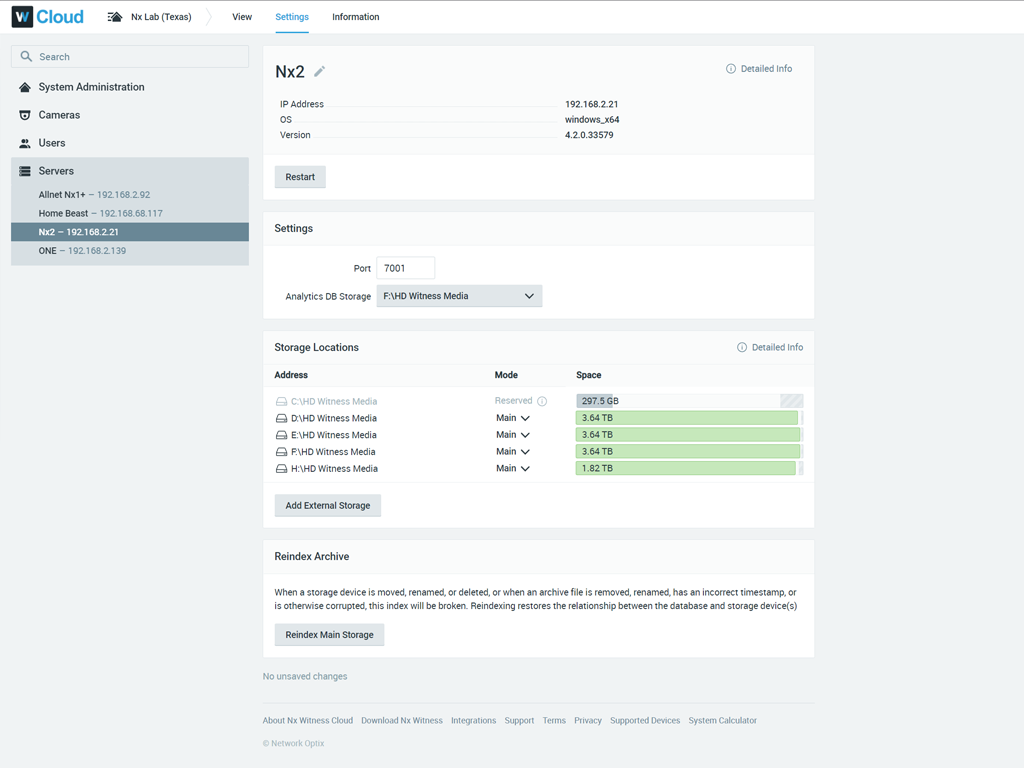Here is the cleaned and detailed caption for the image you described:

---

The image shows a detailed view of a monitoring and control interface from NX Lab, Texas. In the upper left corner, there is a logo within a black box featuring the letter "W" split into two colors—white on the left half and blue on the right. To the right of the logo, the text "W Cloud" appears in blue.

Beneath this, a white header bar displays multiple options: "NX to IP Address," "OS Version," "Detail Info," and "View Settings Information." 

Following the header, the interface is segmented into various sections. The first section titled "NX to IP Address" includes details like the OS version and a restart button. The "Settings" section details configurations such as "Port 7001," "Analytics," "TV," and "Storage HD Witness Media."

Below, the "Storage Locations" section is set against a light gray background with black text, listing different hard drive partitions (E, F, H), with storage capacities running into terabytes (e.g., three terabytes for multiple drives). This section provides precise information about each drive’s storage capacity.

Towards the end, there's another section labeled "Reindex Archive," with a gray button below it. This section outlines procedures and conditions for reindexing the archive, particularly when storage devices are moved, renamed, deleted, or when an archive file has an incorrect timestamp or is otherwise corrupted.

The overall background of the website oscillates between a light gray and a medium-dark gray, providing a clean and organized look to the interface.

---

This descriptive caption outlines each element of the interface and provides a comprehensive overview of the contents and functions available within the image.